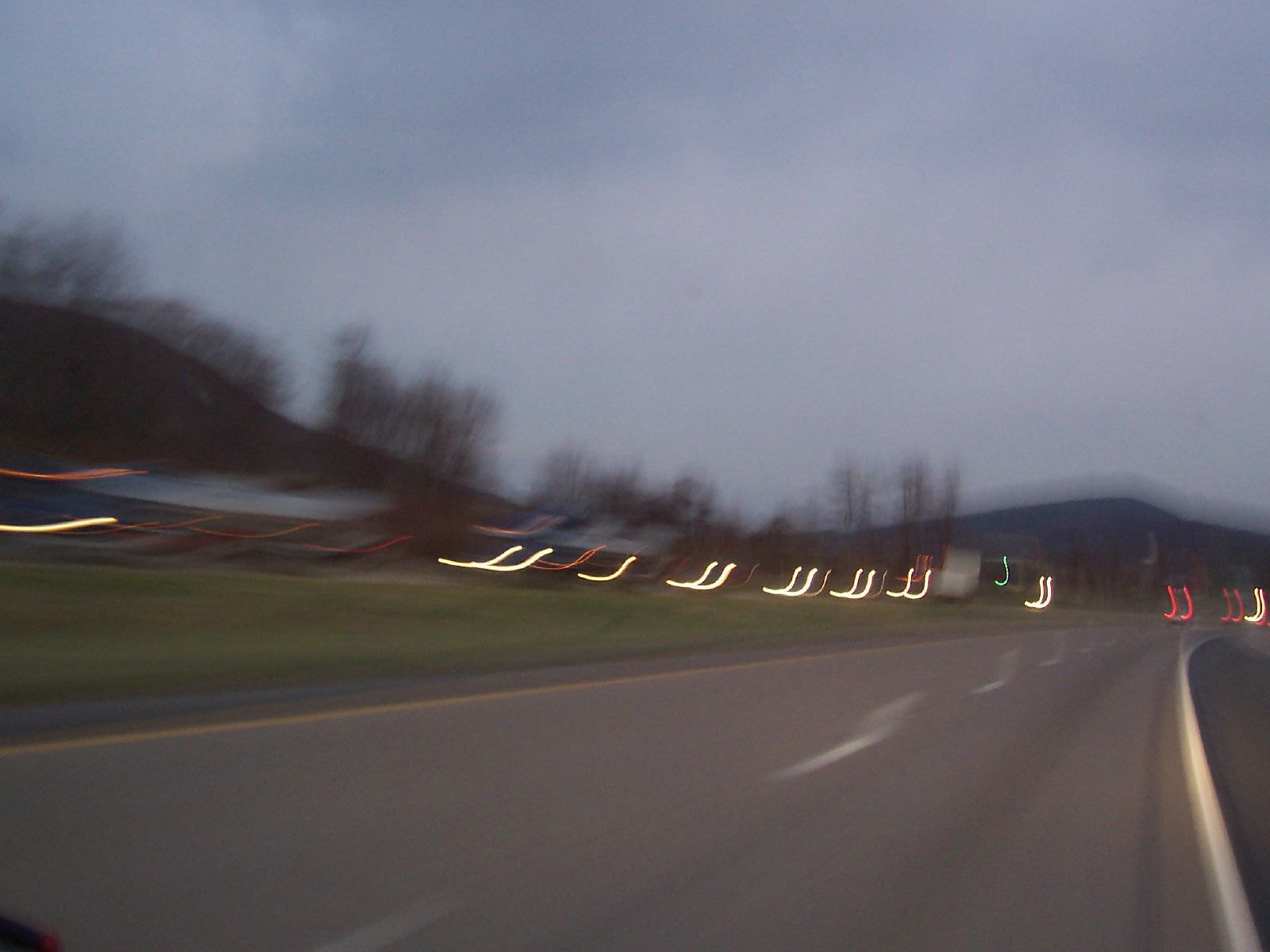This photograph, taken from inside a moving car on a highway, captures a dynamic nighttime scene rich in motion blur. The road, curving to the right, is devoid of nearby cars but is lined with blurred yellow and red lights, creating vibrant, stretched-out streaks in S shapes due to the camera's movement. These light trails include both front headlights and brake lights far ahead, and the dotted center line appears lifted off the ground, adding to the surreal effect. On the opposite side of the median, you can see several sets of oncoming traffic, more numerous than vehicles traveling in the same direction. In the distance, faint red taillights are visible. The landscape features gray-clouded skies, hints of leafless trees suggesting wintertime, and silhouetted hills with some trees, enhancing the chilly, atmospheric quality of the photo.